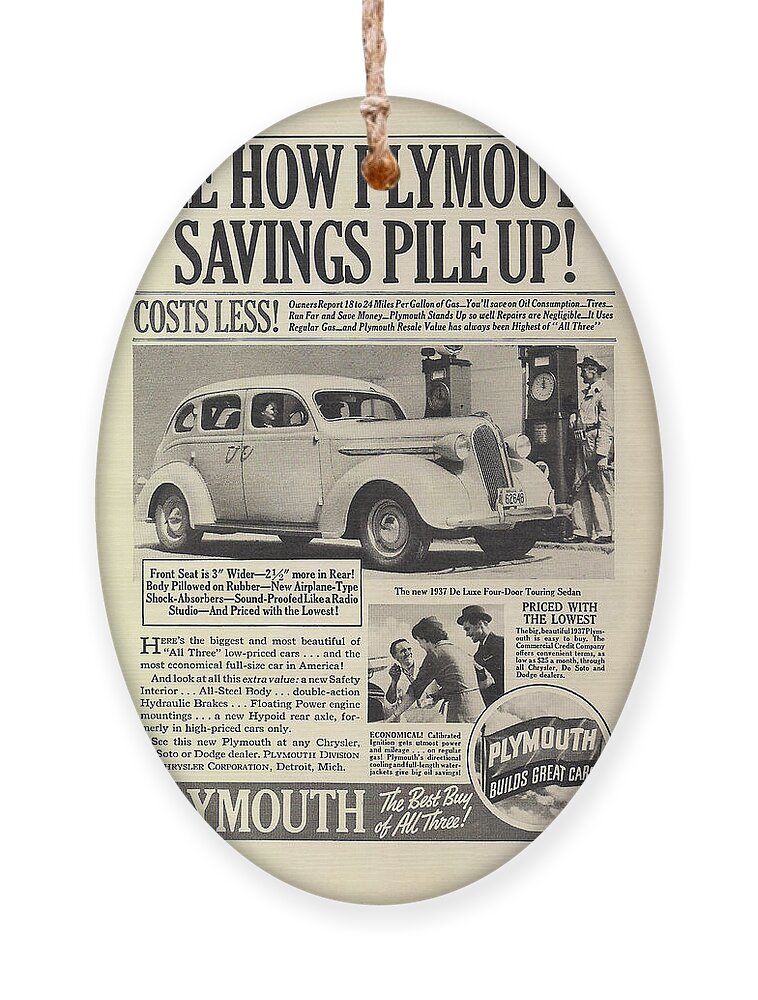The image portrays an oval-shaped hanger with a string looped through a hole at the top, allowing it to hang like a necklace. Inside the oval, there is an old, black-and-white newspaper ad featuring a vintage 1937 Plymouth car. The headline reads "How Planned Miles Savings Pile Up Cost Less," showcasing the vehicle's cost-effectiveness. The advertisement highlights various selling points: 18 to 24 miles per gallon of gas, minimal oil consumption, durable tires, and high resale value. It emphasizes that the Plymouth requires regular gas and boasts a sturdy build with negligible repair needs. Additionally, the ad mentions comfort features such as the front seat being three inches wider, a rear body two and a half inches longer, new airplane-type shock absorbers, and soundproofing comparable to a radio studio. The overall scene is captured against a white background, making the vintage ad the focal point.